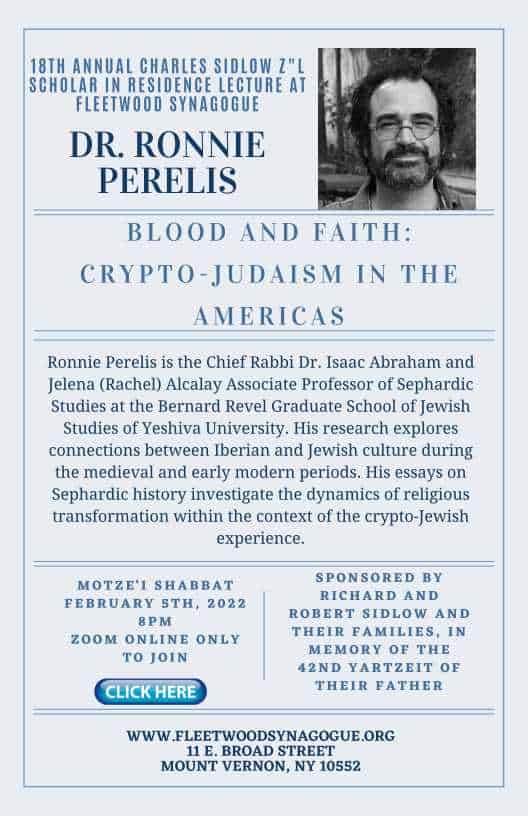This image is a detailed flyer for the 18th Annual Charles Sidlow Scholar-in-Residence Lecture at Fleetwood Synagogue, featuring Dr. Ronnie Perelis. The flyer, outlined in blue on a light gray background, prominently showcases a black-and-white photograph of Dr. Ronnie Perelis, a man in his mid-to-late 40s with a beard, mustache, wire-rim glasses, and dark receding hair, smiling slightly. The text highlights Dr. Perelis’s upcoming lecture titled "Blood and Faith: Crypto-Judaism in the Americas" and provides a brief biography. Dr. Perelis is described as the Chief Rabbi, Dr. Isaac Abraham and Jelena Rachel Alcalay Associate Professor of Sephardic Studies at the Bernard Revel Graduate School of Jewish Studies, Yeshiva University, with research focused on Iberian and Jewish cultural connections during medieval and early modern periods. The flyer indicates the event will be held online via Zoom on Motsae Shabbat, February 5th, 2022, at 8 p.m., with a clickable link to join. It also notes sponsorship by Richard and Robert Sidlow and their families in memory of their father’s 42nd yahrzeit. The footer includes the synagogue’s website, www.fleetwoodsynagogue.org, and its address at 11 East Broad Street, Mount Vernon, NY 10552.